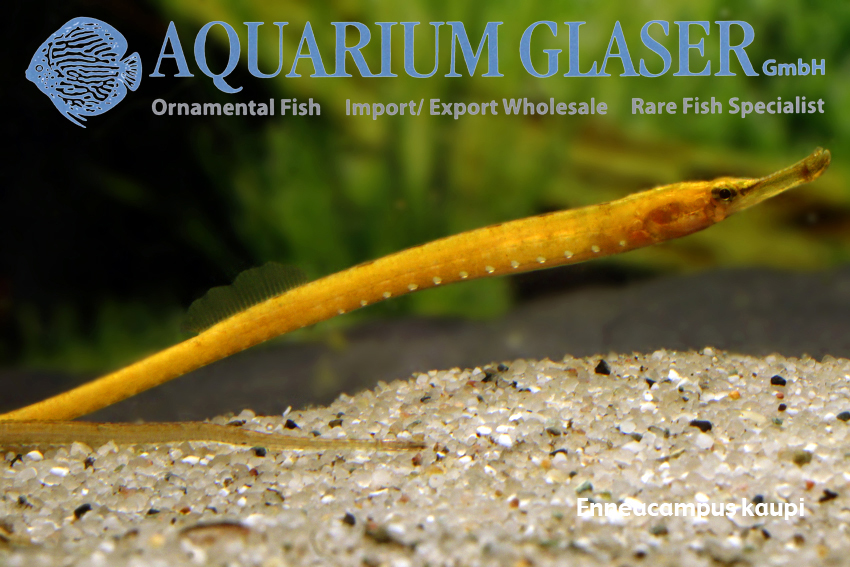This vibrant advertisement for Aquarium Glaser GmbH showcases their expertise as specialists in ornamental fish, emphasizing import-export wholesale and rare species. The centerpiece is a strikingly rare fish, identified as Anayucampus cowpea, depicted swimming gracefully above a sandy bottom that is speckled with white, black, and yellow flecks. The fish, with its long, slender body and distinctive orange hue, features a clearly visible eye and a pronounced long snout on the right-hand side. The backdrop consists of a green, seagrass-filled aquarium setting, enhancing the exotic nature of the fish. At the top of the ad, the store's logo is prominently displayed, featuring a big blowfish alongside the name "Aquarium Glaser GmbH" in blue text. Adjacent to this, the tagline emphasizes their status as rare fish specialists.